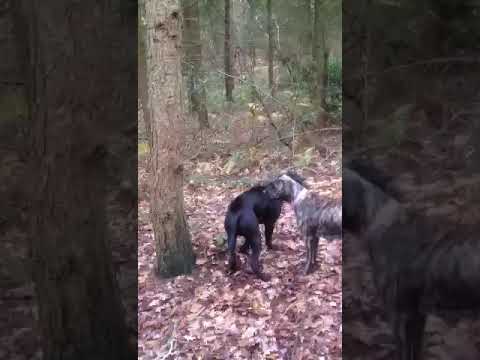A vertically aligned, low-resolution photograph captures a blurry, overcast scene in a forested area. The image, flanked by thick black bars on either side, primarily showcases an expanse of fallen leaves in shades of brown, red, and yellow, carpeting the ground in the bottom half. The terrain appears to be on a slope, indicating a subtle incline. In the top half of the photo, numerous tree trunks extend upwards, with a mix of deciduous and evergreen trees stretching into the distance. Sparse green leaves and shrubbery dot the landscape amidst the trunks. Light filters gently through the branches, hinting at a daytime setting.